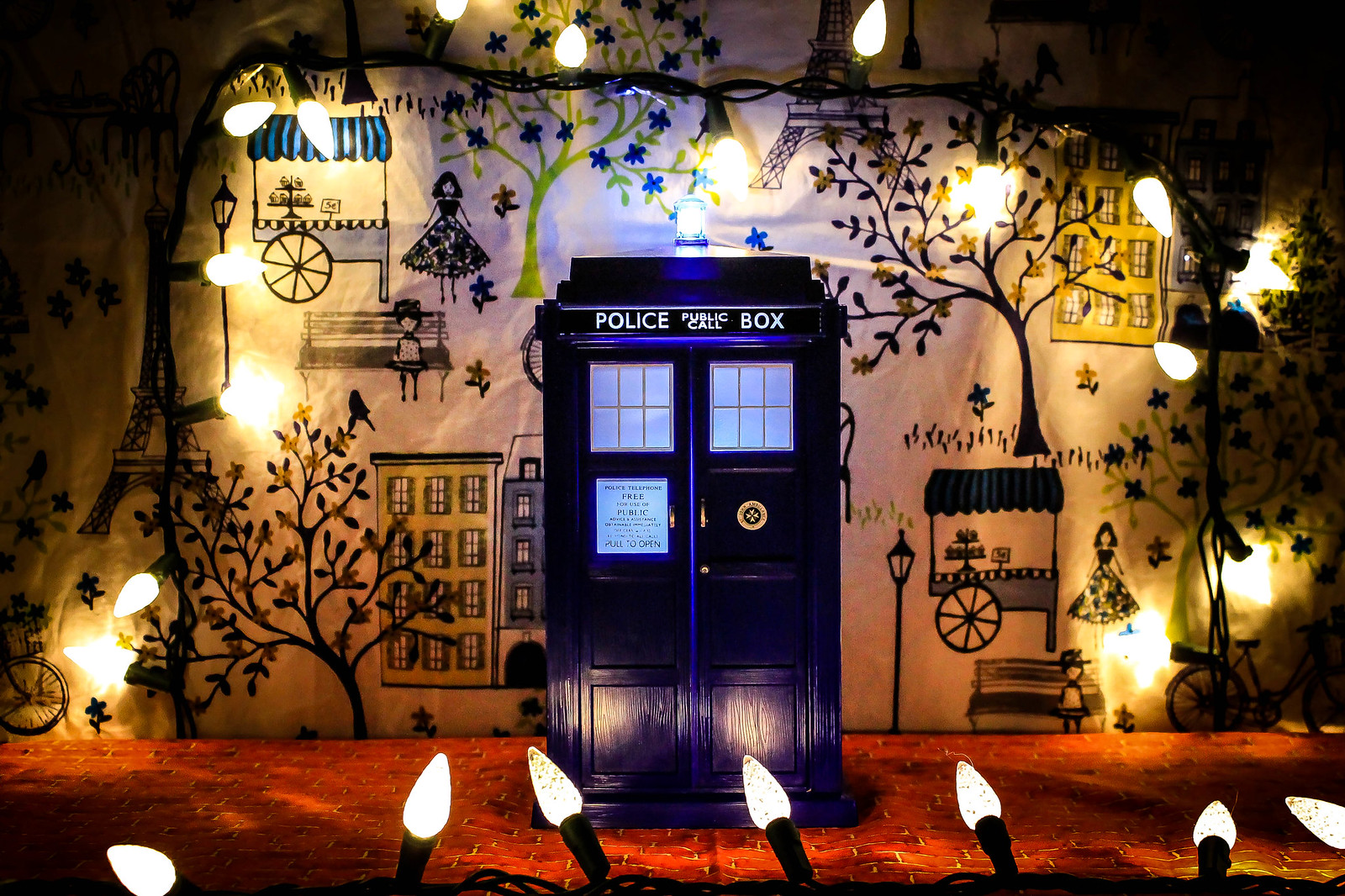This detailed color photograph captures a play stage featuring a central prop designed as a police public call box, prominently labeled at the top. The dark blue, rectangular box has two doors with windows, and a small blue sign with unreadable text below the left window. The box rests on a brick-patterned floor, surrounded by illuinated white lights, resembling Christmas tree lights, framing the scene. The backdrop consists of a hand-painted cityscape on white fabric, depicting various urban elements in black, yellow, and blue hues. To the left of the call box is a tall building with numerous windows, while to the right is a vendor's cart with a woman standing beside it. Further in the background, there are trees, another cart with a woman nearby, a bench with a boy sitting, and a yellow building with white windows. The edges of the image appear dark due to insufficient lighting, enhancing the dramatic effect of the illuminated stage.